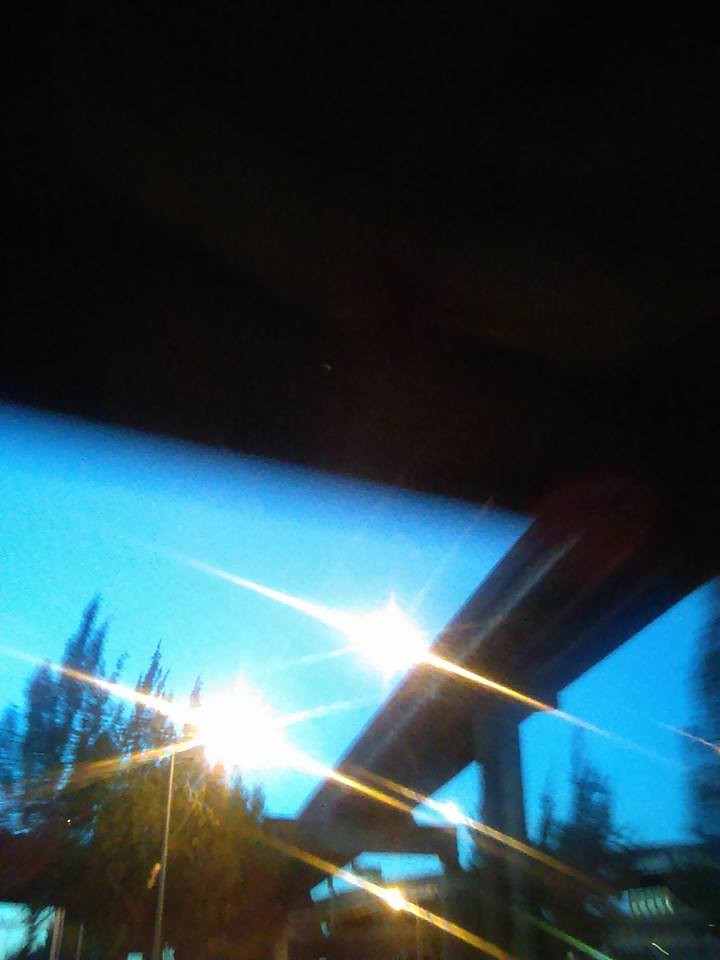The photograph, taken from inside a moving car, captures a blurry and grainy scene dominated by a striking, dark arc overhead which appears to be an elevated railway track extending towards the background and away from the viewer. Below this dark structure, two street lamps shine brightly, their rays creating lens flares that streak across the blue sky, which is clear and devoid of clouds. In addition to the railway bridge, there's another bridge below it that extends off to the right. To the left of the scene, a small wooded area with dense, leafy trees is visible. The reflection of sunlight on the car's windshield adds to the glare and overall haziness of the image, contributing to its dreamlike quality.